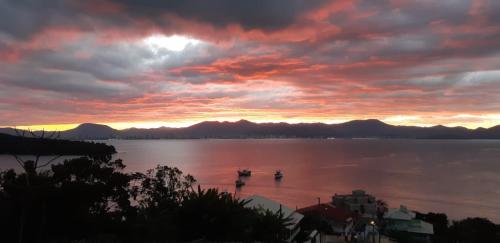This small, horizontal rectangular image captures a tranquil sunset scene viewed from an elevated vantage point. The centerpiece is a serene lake, its glassy surface casting a reflective, reddish hue from the vibrant, setting sun. Scattered across the water are three small, indistinguishable objects—likely boats, although they could also be boulders protruding from the lake's surface. 

In the foreground, silhouetted trees with visible leaves stretch along the left side, creating a dark outline against the colorful backdrop. The land in the lower left corner reveals indistinct structures—a few buildings, one with a white roof, another multi-level, and possibly a house. To the right, additional silhouettes of houses are barely discernible due to the dim lighting. 

The distant background features a range of dark, hilly terrain bordering the lake. Above, the sky is a breathtaking spectacle with high clouds painted in shades of pink, blue, red, purple, and gray. Near the horizon, a small, bright circle of sky peeks through the clouds, casting an almost magical light that enhances the serene, reflective quality of the scene. The dark silhouettes combined with the vivid sky and smooth, reflective lake create an image that is both atmospheric and contemplative.